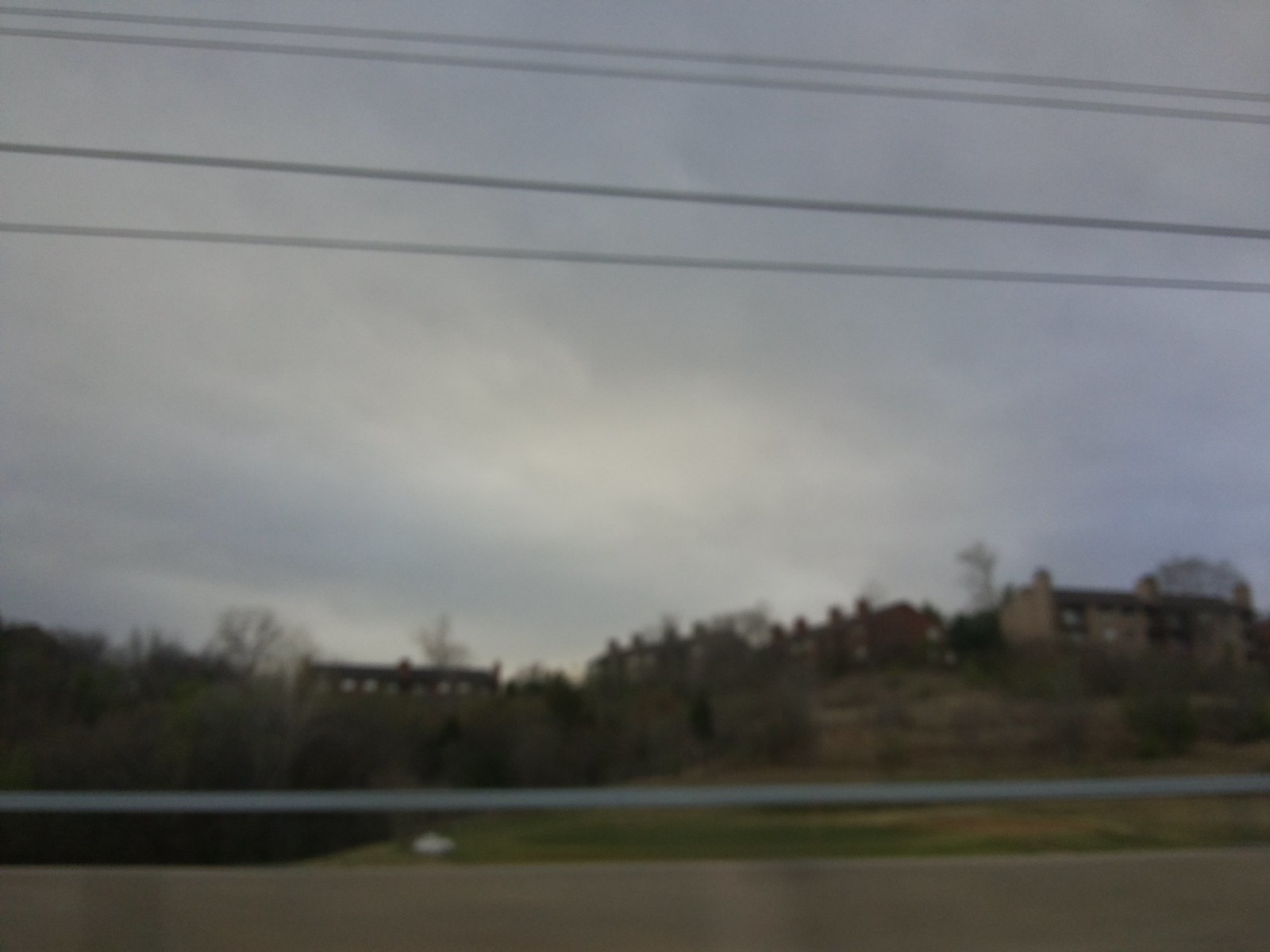A blurred photograph captures a scene from a moving vehicle, revealing a highway and adjacent service road. A guardrail runs alongside the road, while to the right, building structures stand atop a knoll. A hillside speckled with shrubs and hedges stretches out beneath an overcast sky. Overhead power and utility lines trace their path along the roadside. The overcast day lends a dim and muted tone to the image, with bushes and trees softly fading into the background. The motion of the vehicle is evident, lending a dreamy, unfocused quality to the entire scene.